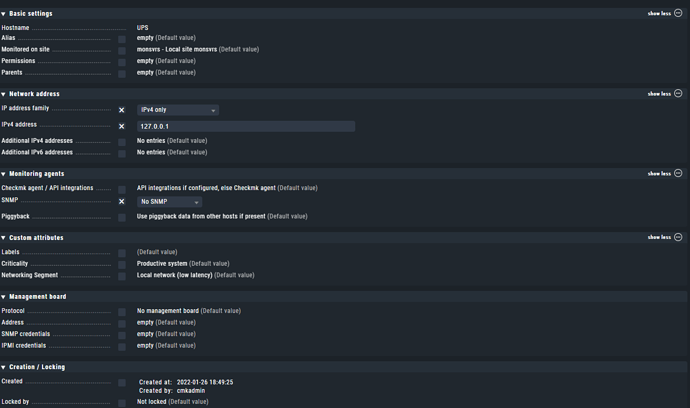This screenshot displays a black interface with sections of white text, presenting a series of settings and options likely related to a software application or web service. The text is particularly small, making most of the words difficult to decipher. Key visible terms include "Basic Settings," "UPS," "Empty," "Moderators," "iPad Only," "No Entries," and "API Registration." Additionally, the screen contains various references to agents, guidelines, and locking mechanisms. The presence of numbers suggests elements like phone numbers or IP addresses. The layout of the screen is divided into distinct sections, but the minute font size renders the majority of the text indistinguishable, leaving the overall context of the screenshot unclear.